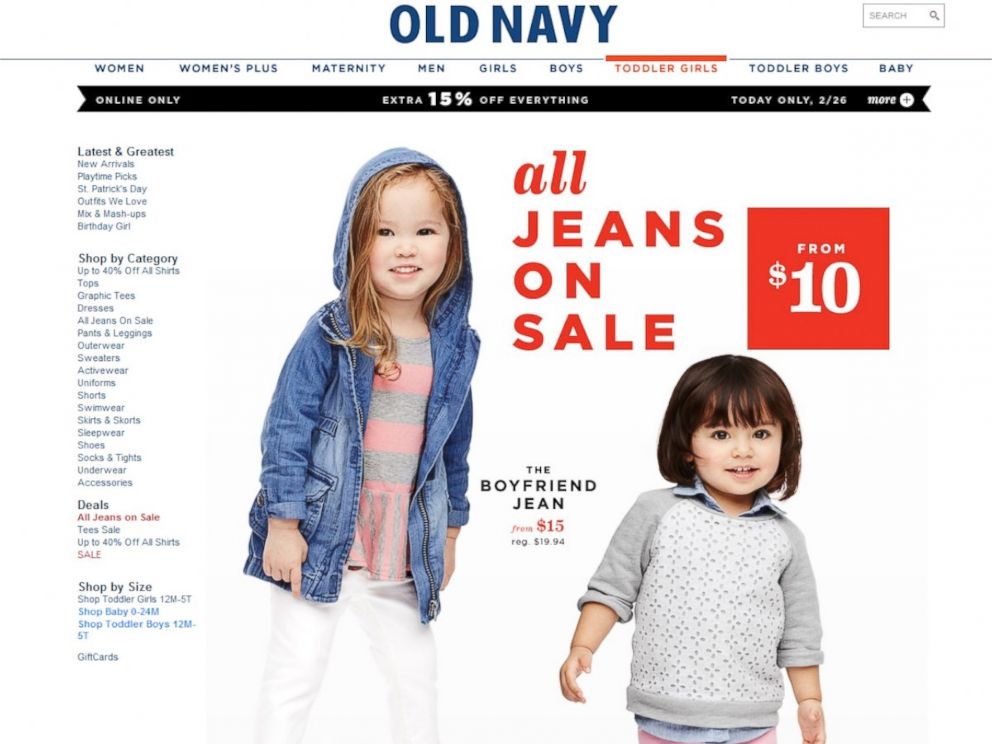The webpage displays the Old Navy website, with a clean and organized layout. At the top center, the Old Navy logo is prominently featured in blue. Directly beneath this, a horizontal menu lists various categories in blue: Women, Women's Plus, Maternity, Men, Girls, Boys, Toddler Girls, Toddler Boys, and Baby, with the Toddler Girls category highlighted in red, accompanied by a red underline, indicating a special focus or promotion in that category.

In the main section of the page, a charming image features two young children. On the left, a smiling girl who appears to be around five years old stands slightly sideways. She is dressed in a stylish jean jacket with a hood, layered over a pink and gray striped shirt. On the right side of the image, a young boy is wearing a cozy gray sweatshirt with a contrasting white body adorned with a subtle gray design pattern.

Text overlays between the children promote "the boyfriend jean from $15, regular $19.94," written in small black letters. Just above this text and to the right, highlighted in red letters, is the phrase "all jeans on sale." Above the boy's head, a red square with white text advertises jeans starting "from $10."

On the left side of the page, there is a vertical menu offering additional browsing options. Categories include "latest and greatest," "St. Patrick’s Day outfits we love," and more. Visitors can shop by specific categories including outerwear, sweaters, uniforms, and shorts. The menu also highlights current deals such as "all jeans on sale," and a section to shop by size.

Directly beneath the top horizontal menu, a black bar spans the width of the page, bearing the notice in white text: "online only extra 15% off everything. Today only 2/26."